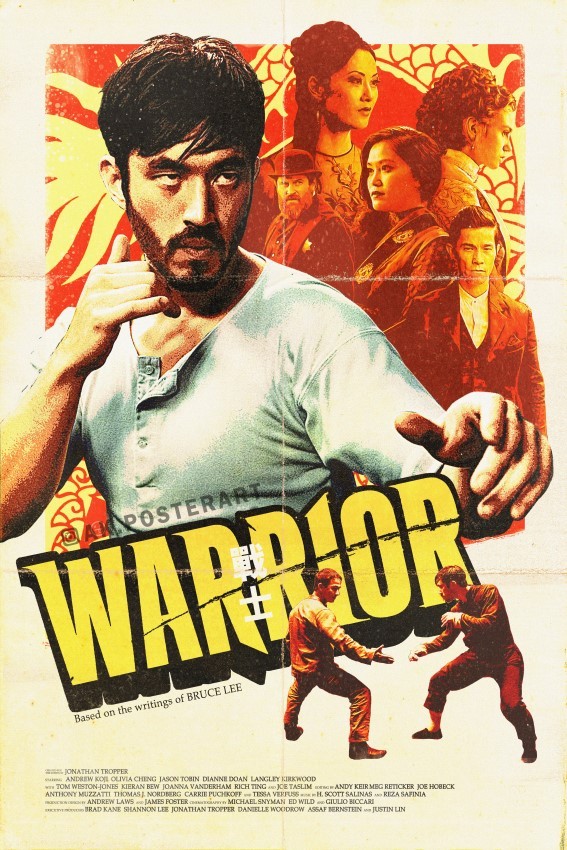This is a vintage-style movie poster for the film "Warrior," based on the writings of Bruce Lee. The poster, showing signs of age with visible creases and wear along the edges, features a central figure who doesn’t resemble Bruce Lee but has a mustache and beard, standing in a fighting stance. The man appears to be Asian, wearing a short-sleeved, collarless white shirt. Behind him is a montage of various characters, including two Asian women with long hair, one with braided and the other with straight hair, a red-headed, bearded man in a bowler hat, an Anglo-looking woman, and a young man with a narrow face in a suit and tie. 

The background of the top part of the poster is patterned with a gold and red dragon motif. The title "Warrior" is prominently displayed in yellow letters with a black outline, overlaying a white symbol, and above it is a watermark reading "AM poster art." Below the title, the text reads "Based on the writings of Bruce Lee." The lower part of the poster has a cream-colored background with detailed movie credits, typical of a traditional movie disc cover.